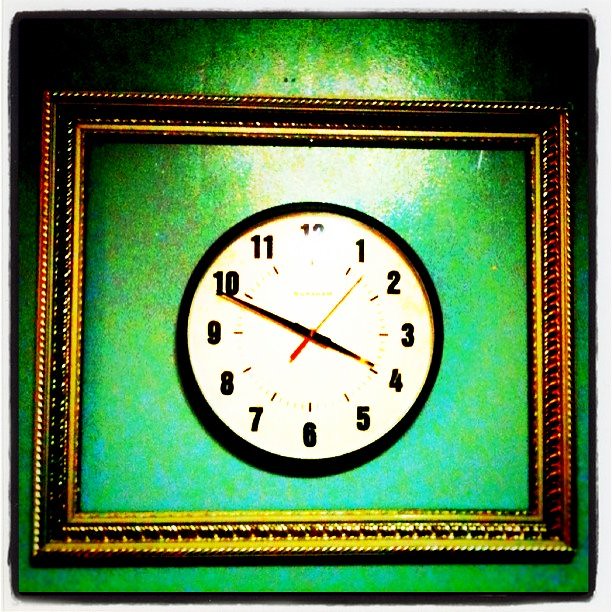This intriguing image captures a clock that is beautifully framed and mounted on a striking jeweled green wall. The frame itself is an elaborate, golden structure that significantly oversizes the clock, drawing attention to the artwork-like presentation. The clock, resting at the center of this large, ornate frame, is a traditional circular design with a black outer rim and black numerals. The clock face shows the time as approximately 10 minutes to 4, with a red second hand positioned between the numbers 1 and 2. A camera flash has been used to capture the image, causing a reflective glare that obscures the bottom part of the number 12 and casts a gleaming highlight on the wall above the clock, adding an unexpected and fascinating effect to the composition.